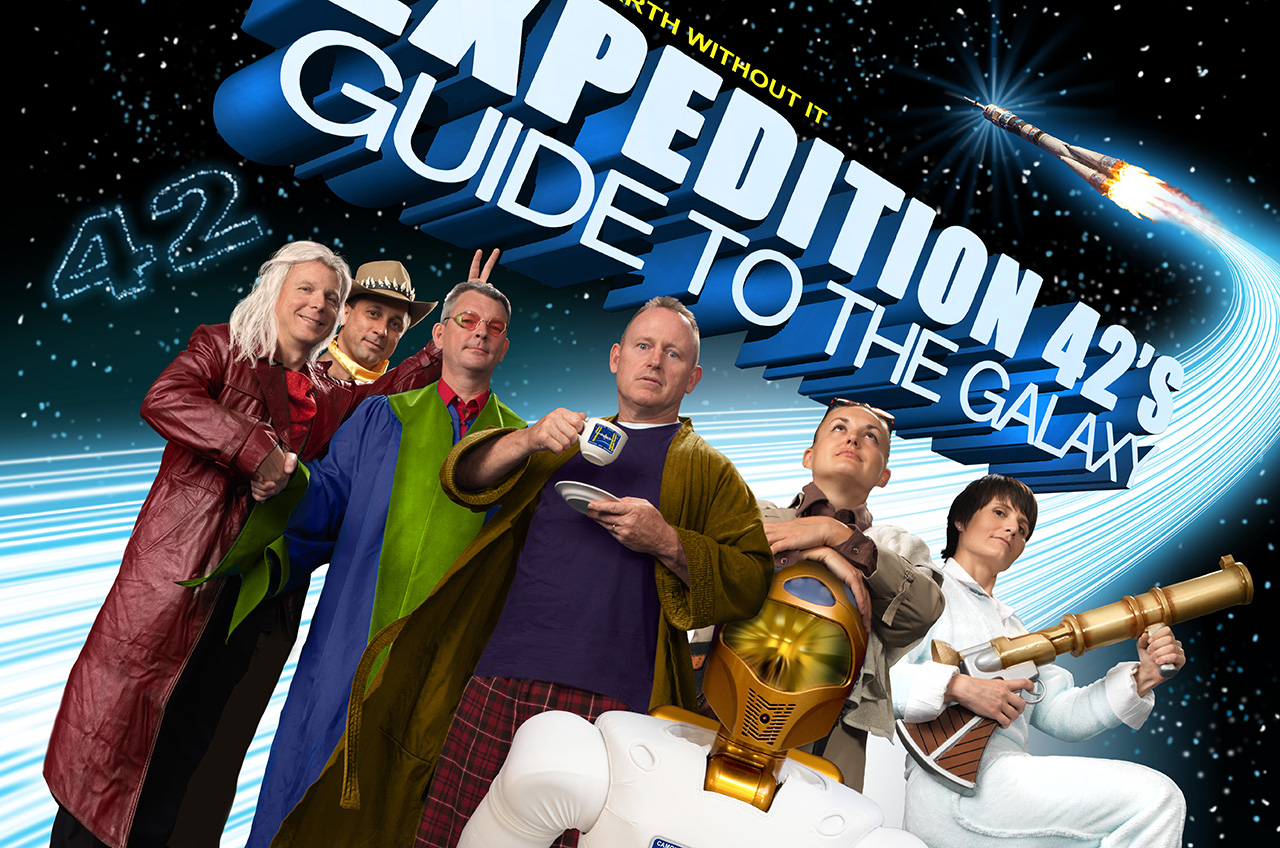The image depicts a detailed and vibrant promotional poster for the TV production titled "Expedition 42's Guide to the Galaxy," which draws inspiration from the Hitchhiker's Guide to the Galaxy. The poster is a colorful and intricately designed blend of realism, photographic representationalism, and graphic design. 

The title "Expedition 42's Guide to the Galaxy" dominates the top portion of the image, inscription at an angle from the top left towards the middle right, showcasing 3D muted blue typography with a wide 3D effect. Directly below the title, at a downward slant, are six cast members positioned diagonally, each donned in their unique costumes from the production. 

One of the main characters, centrally located, is depicted holding a teacup with a matching small plate, exuding a significant presence. To the bottom right of the cast, an android-like creature stands out, adorned with a gold and white mask that forms part of its design. In the upper right corner, a space rocket is seen, its path illuminated by a trail of light blue and white streaks, indicating a dynamic motion through space.

The background sets a cosmic stage with a star-lit black expanse. The number "42," formed by a constellation of stars, appears prominently on the upper left side. Various shades of green, blue, gold, copper, white, brass, gray, burgundy, black, and light blue add to the rich visual tapestry of the scene. The poster effectively conveys the sci-fi theme and adventurous spirit of the series, capturing the essence of an intergalactic expedition.